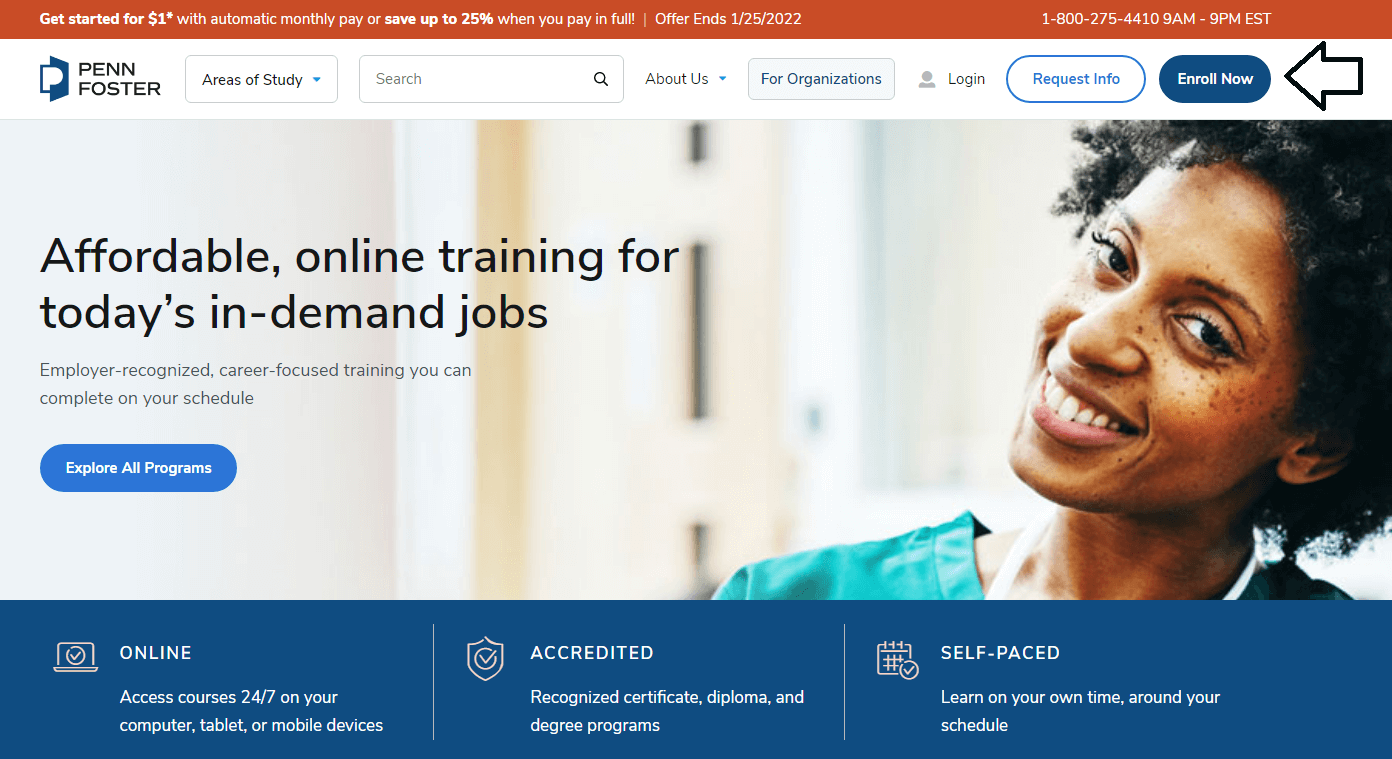The image is a left-to-right horizontal layout, sourced from a website accessible via a computer or a smart device. At the top of the image is a small, long horizontal orange rectangle featuring a promotional text in white: "Get started for $1* with automatic monthly pay or save up to 25% when you pay in full. Offer ends 1-25-2022." To the right of this is the phone number and service hours, listed as "9 a.m. to 9 p.m. Eastern."

Moving further to the right, the banner showcases the Penn Foster logo along with several navigational links, including "Areas of Study," a search bar, "About Us," "For Organizations," a "Login" button, "Request Info" in blue, and "Enroll Now" in navy blue with an arrow pointing to the button.

Below the navigational banner is a photograph of an African American woman. She is smiling, and the image captures her from her top neck and head. Adjacent to this photograph, the text reads: "Affordable online training for today's in-demand jobs. Employer-recognized career-focused training you can complete on your schedule." Below this text is a button labeled "Explore All Programs."

Towards the bottom of the image, there is a navy blue section featuring several icons and descriptive text blocks. The sections are titled "Online," "Accredited," and "Self-Paced," each accompanied by a brief explanatory blurb.